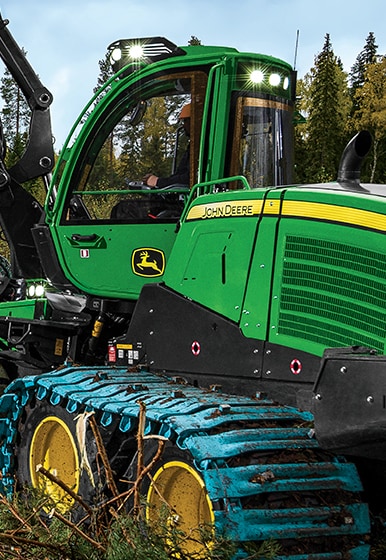The image showcases a large and imposing John Deere all-terrain vehicle, prominently featuring the brand's iconic bright green and yellow colors. The cab of the tractor is painted in green, adorned with the yellow and black John Deere logo near the door and a yellow stripe along the rear side, clearly marking it as a John Deere machine. The tires are yellow and black, with teal-colored conveyor belt-like coverings that suggest its capability for rugged terrain. A man is visible inside the cab, operating the vehicle. The vehicle's lights are on, and a black, hook-like appendage extends skyward from the machine, which could be used for digging. The backdrop consists of tall, dark evergreen trees set against a blue-gray sky with some light clouds, adding depth to the rural scene. On the ground in front of the tractor, there's a mix of brush, sticks, and green leaves.